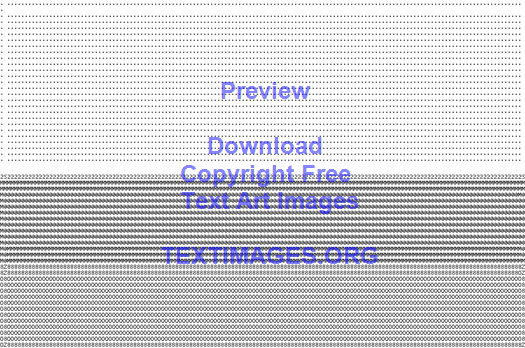The image from textimages.org is a rectangular graphic featuring a variety of black letters and numbers arranged horizontally across the page. At the top, the spacing between the characters is sparse, but it becomes denser toward the bottom, eventually filling the space with greater textual density. In the top portion of the image, blue-colored text displays the word "Preview". Below it, there are successive lines of text that read "Download", "Copyright Free", and "Text Art Images". At the very bottom, also in blue, the URL "textimages.org" is prominently featured. The overall appearance of the background resembles patterns created by various letters and numbers, contributing to a visually dense textual art piece that adds a unique decorative element to the image.